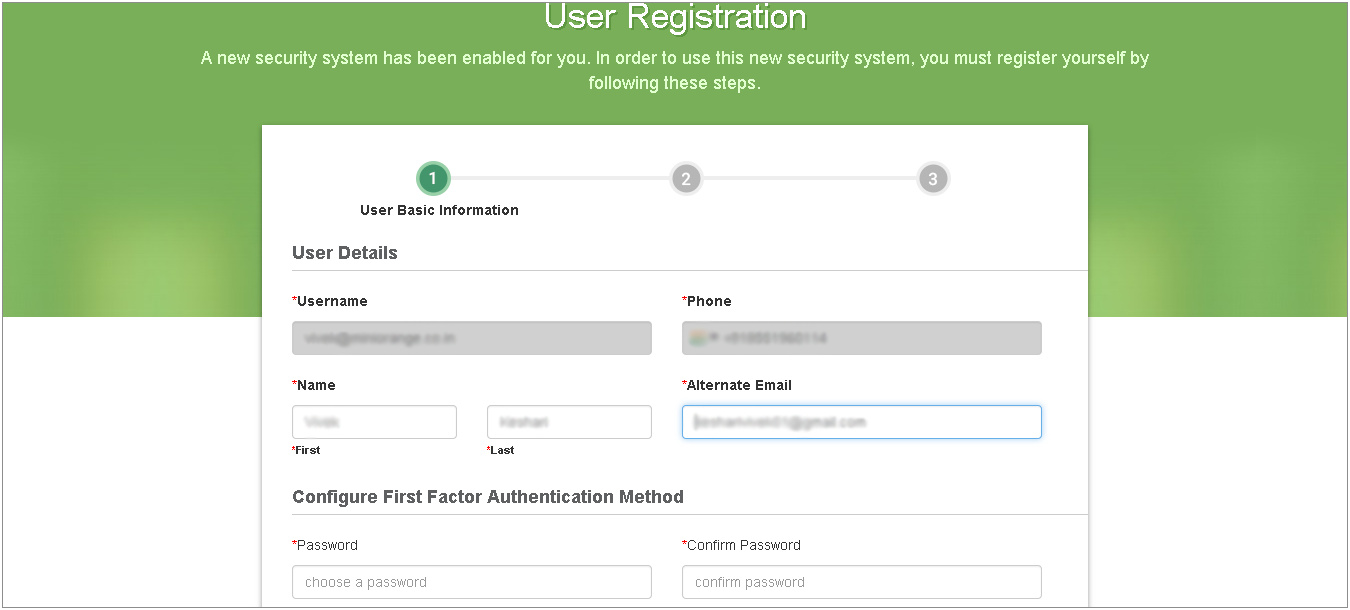The screen displays a user registration webpage with a green header and a white background. The header reads "User Registration," accompanied by a notification indicating that a new security system has been enabled. To use this system, users must complete the registration process by following a series of steps.

Step one, highlighted in green, requires users to provide basic information. Subsequent steps two and three are greyed out. 

The form under step one includes several fields:
- **Username:** Marked with a red asterisk, accompanied by a text box for input.
- **Phone:** Also marked with a red asterisk, with a corresponding text box.
- **Name:** Comprising two text boxes, one labeled "First," the other "Last," both marked with red asterisks.
- **Alternate Email:** With a red asterisk, followed by a text box for entry.

Further, users are required to configure their first factor authentication method:
- **Password:** Marked with a red asterisk, accompanied by a text box.
- **Confirm Password:** Also marked with a red asterisk and followed by a matching text box for re-entering the password.